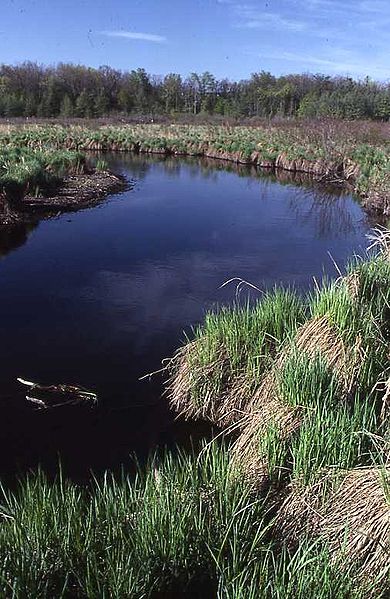This is a detailed photograph of an outdoor landscape, featuring a narrow, winding body of water that appears to be either a creek or the edge of a pond. The water curves to the left and forks off, disappearing into the marshland, where dense green and brown grass surrounds the banks on both sides. The water itself is a dark bluish color with a hint of clarity, and floating grass and possibly some dead vegetation are visible on its surface. In the foreground, more thick grass can be seen, extending into the distance. The scene is complemented by a heavily wooded area in the background, with an array of trees whose specific types remain indiscernible. The sky overhead is blue with light cloud cover, suggesting a clear day with moderate sunlight. There are no people or textual elements in the image, giving it a serene, undisturbed quality. A distinct piece of grass or some small object floats in the water near the bottom of the image, adding a subtle point of interest.